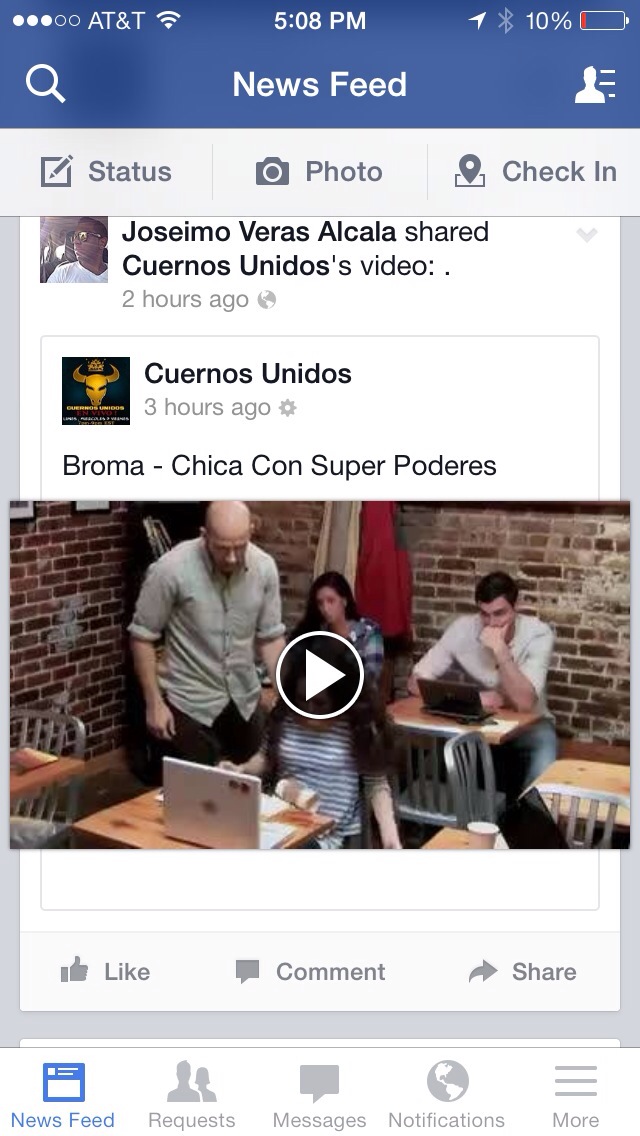The image is a detailed screenshot from an iOS device, specifically an iPhone, displaying the Facebook application. At the top left corner, the carrier is identified as AT&T, while the top center shows the time as 5:08 p.m. and the right side indicates a 10% battery status. Directly below, a blue bar reads "News Feed," accompanied by a magnifying glass search icon on the left and a profile avatar icon on the right. Underneath this blue bar, there's a gray tab bar with options "Status," "Photo," and "Check-in."

The main body of the screenshot highlights a Facebook post from Josima Veras Alcala, who shared a video originally posted by "Suerna's Unidos." The thumbnail of the video depicts people in a cafe with laptops. Below this post, user interaction options "Like," "Comment," and "Share" are visible. Finally, at the bottom of the screenshot, the Facebook navigation bar is present with icons and labels for "News Feed," "Requests," "Messages," "Notifications," and "More."

The color scheme includes various shades such as blue, white, gray, black, yellow, dark blue, brown, red, green, and gold, rendering it visually rich. The overall layout clearly identifies it as a Facebook interface on an iPhone screen.